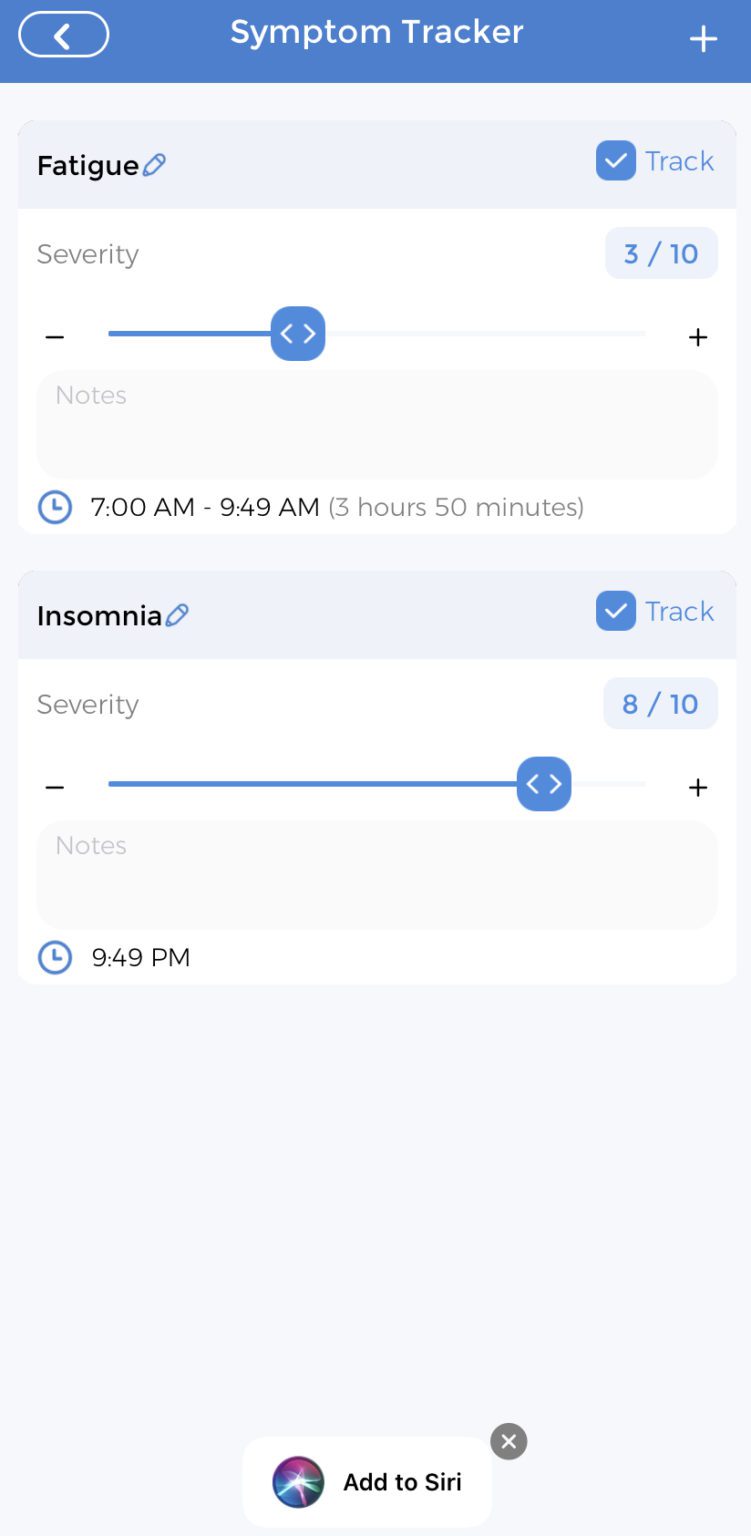A screenshot of a symptom tracker app displays a detailed log of two symptoms: fatigue and insomnia. 

- **Fatigue**:
  - Severity: 3 out of 10
  - Edit option: Represented by a pencil icon
  - Tracking time: 7:00 AM to 9:49 AM (3 hours and 50 minutes)
  - Notes section: Empty

- **Insomnia**:
  - Severity: 8 out of 10
  - Edit option: Represented by a pencil icon
  - Tracking time: 9:49 PM
  - Notes section: Empty

The overall background of the app is a light blue color. 

At the bottom of the screen, there's an icon resembling thunder or lightning, and an option to "Add to Siri" within a white triangle containing black text. Just above it, there is a gray circle with a white 'X' in the center.

The top bar features a left-pointing arrow on the left side and a plus sign on the right side.